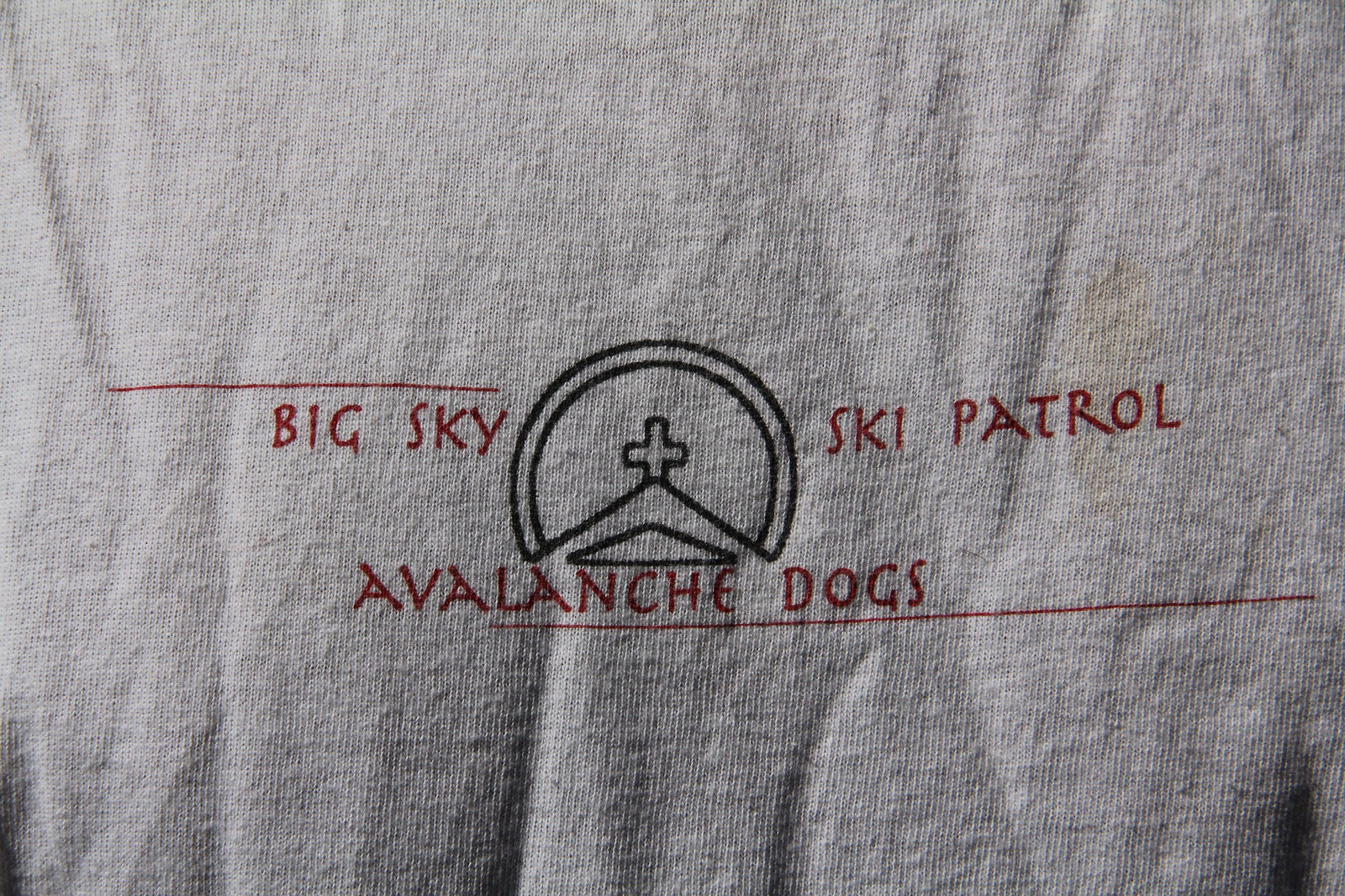This is an extreme close-up image of a heather grey, wrinkled t-shirt adorned with a minimalist, wide logo featuring the text and graphics in red and black. The t-shirt has a faded appearance with a noticeable food stain over "Patrol" on the right side. The logo reads "Big Sky Ski Patrol Avalanche Dogs" with detailed placements: 

- "Big Sky" is on the left, accompanied by a thin red line above it.
- The center showcases a black graphic—a cross on a hill within a semi-circle.
- "Ski Patrol" appears to the right of the graphic.
- "Avalanche Dogs" is centered at the bottom with a line extending from the "L" in "Avalanche" to the far right edge of the shirt.
  
Overall, the design is straightforward and functional with distinct, clean lines.